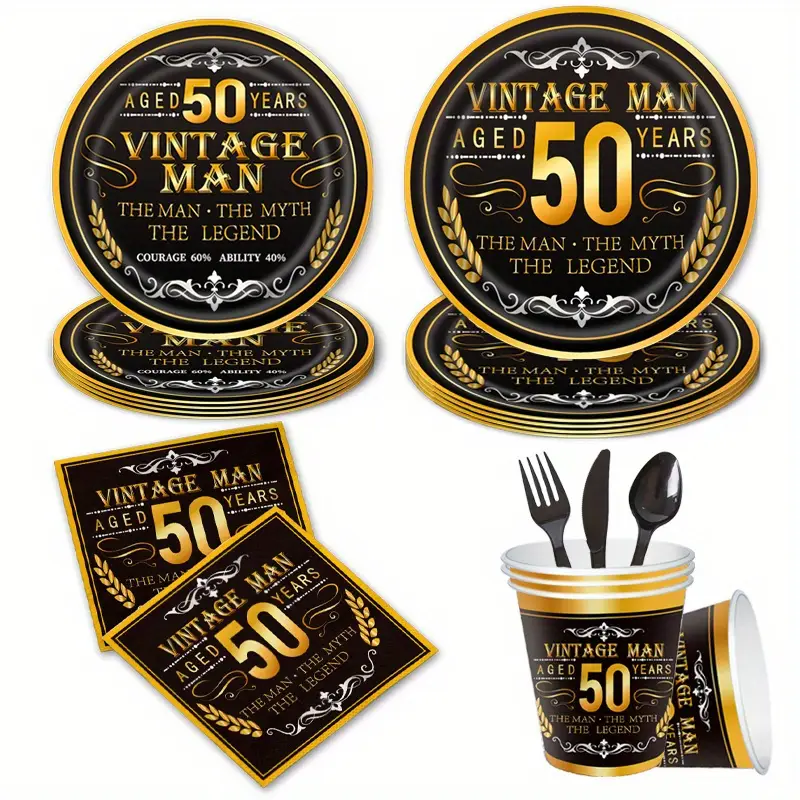The image displays a party-themed setup for a 50-year-old celebration, featuring an array of matching paper products and utensils. At the center, the paper plates are predominantly black with a gold rim. In the center of the plates, gold lettering reads "Age 50 Years Vintage Man," followed by "The Man, The Myth, The Legend." A touch of elegance is added with gold leaves flanking these words. Complementing the plates, the paper cups share the same design and inscription, with their interiors colored black. For dining, a black plastic fork, knife, and spoon are neatly placed within the cups. Additionally, identical napkins with the same black and gold motif are displayed, echoing the plates' and cups' design. All the products, including the napkins, are part of a cohesive set, likely meant to be showcased in advertisements or online stores. The overall color palette of black and gold exudes a sophisticated and celebratory vibe, perfect for highlighting the milestone of reaching 50 years.